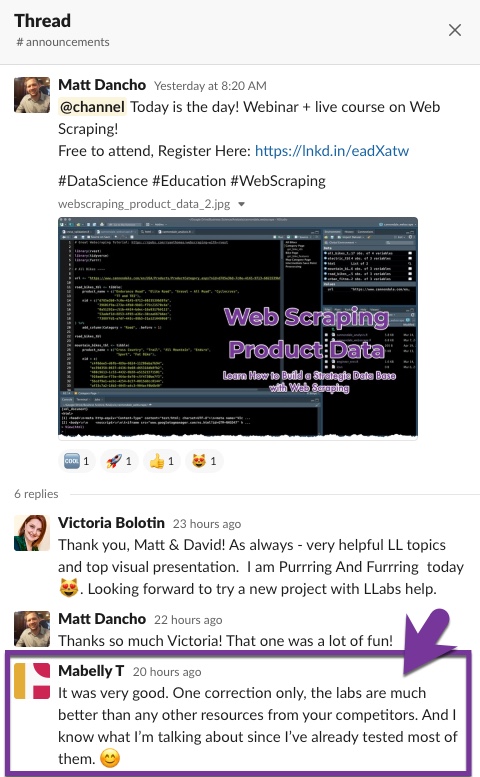**Detailed Descriptive Caption:**

The image showcases a social media post on a white background with black text prominently displaying the word "Thread." On the right side, there is a grey 'X' icon indicative of a close option. The post is tagged with "#announcements."

Posted by Matt Doncho yesterday at 8:20 AM, the message is associated with his profile picture. His photograph, framed in a square, features a smiling man wearing a button-down shirt. The content of his post reads: "Channel, today is the day! Webinar plus live course on web scraping. Free to attend, register here." A blue hyperlink directs users to LinkedIn. Additional hashtags included are #data science, #education, and #web scraping.

Below the main text, a screenshot of the webinar program is visible. The screenshot has a predominantly black background with blue and purple elements and displays the title "Web Scraping Product Data."

Interactions with the post are evident: emojis such as a kitty, a thumbs up, and a rocket, indicating various reactions, are present. There are six replies, one of which is from Victoria Bulletin. Her profile image features a woman with red hair smiling. Her response reads: "Thank you, Matt and David, as always very helpful, LL Topics and top visual presentation. I am purring and furring today," followed by a cat emoji with hearts. She adds, "Looking forward to trying a new project with LL Labs today."

The engagement indicates a positive and active community response to the announcement of the webinar and live course.